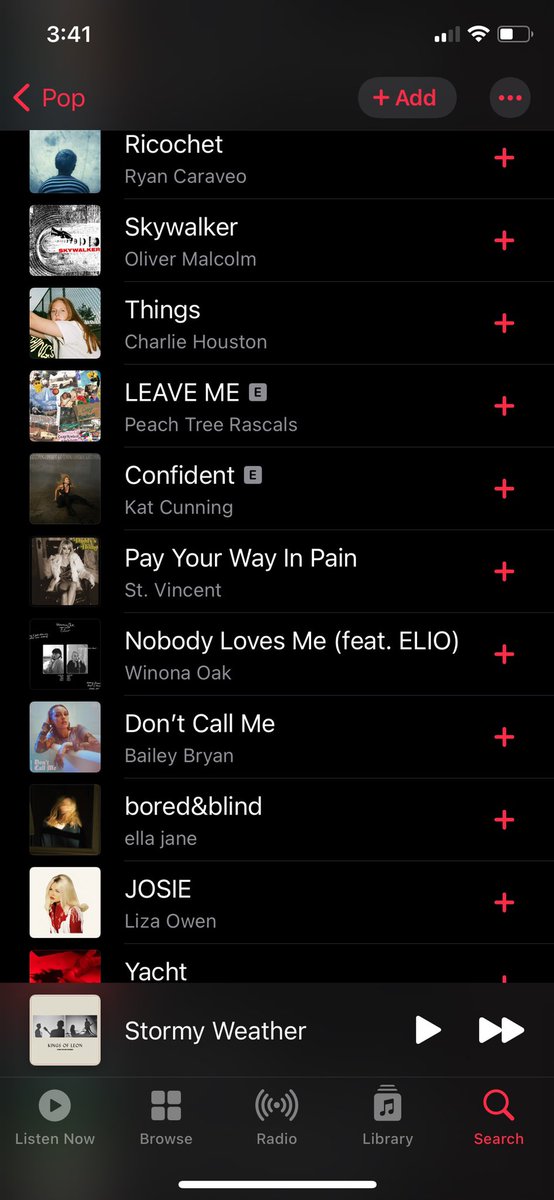A screenshot of a music app interface on a smartphone, captured at 3:41 PM. The device's Wi-Fi signal is strong with two out of four bars, and its battery level is around 50%. At the top of the screen, the genre "Pop" is highlighted in red, indicating the current playlist. There's a red arrow allowing the user to navigate back and possibly select another genre. The playlist is visible with twelve songs listed, and a plus icon at the top enables the user to add more songs. A three-dot menu is present, though its function is unspecified.

The currently playing song is "Stormy Weather," displayed with an album cover that is predominantly white with a black and white center, although the artist's name is not discernible. Playback controls are situated at the bottom, including a play button (single arrow) and a skip button (double arrows).

At the very bottom of the screen are the navigation options: "Listen Now," "Browse," "Radio," "Library," and "Search." The "Search" icon is highlighted in red, suggesting that either a search has been conducted or the user is poised to search.